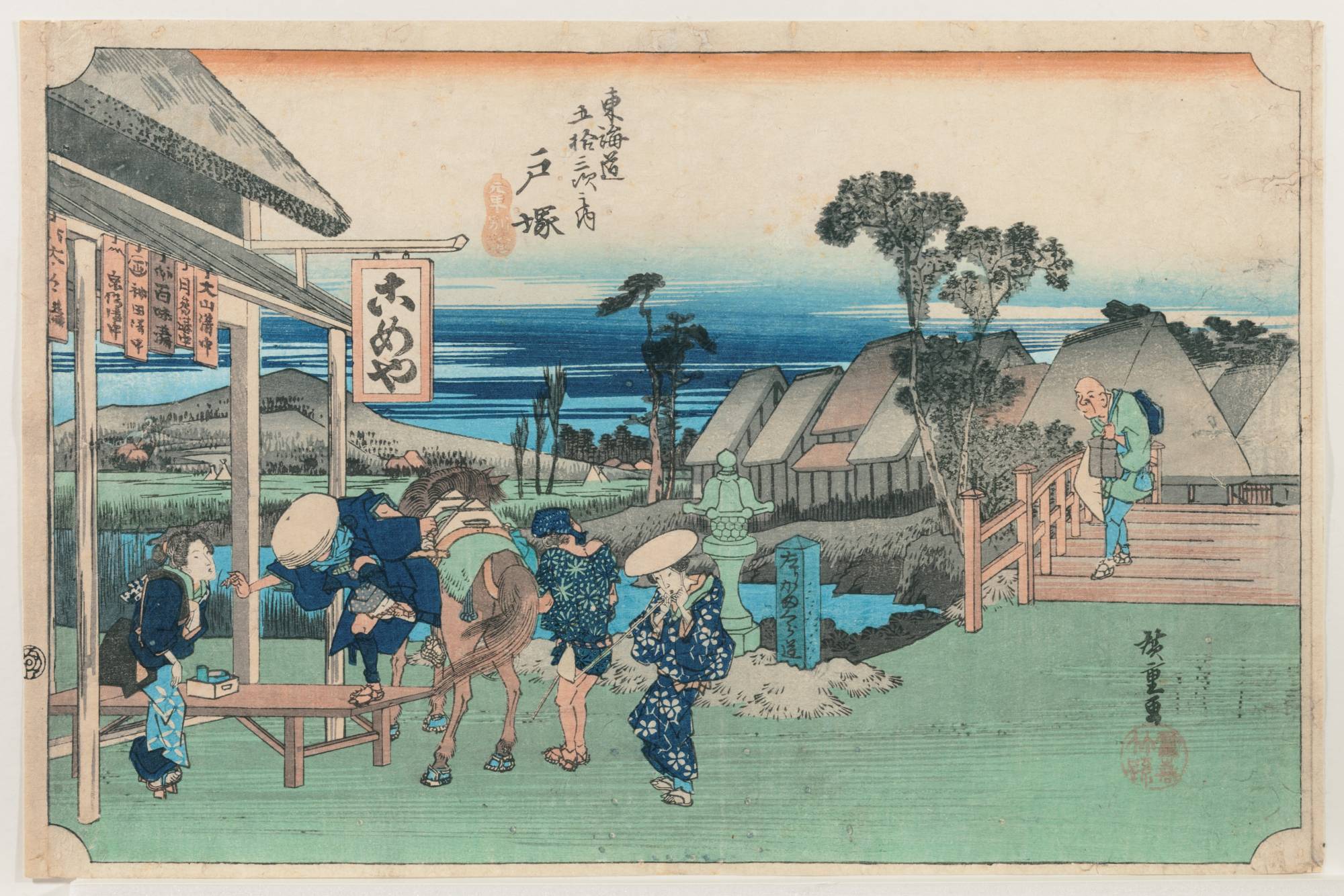This illustrated print, rendered on ivory-toned, slightly aged and dirty paper, captures a traditional East Asian scene—possibly Japanese or Chinese. Dominating the left side of the image, a pagoda-style house features a gray roof and white columns, with decorative elements hanging off the roof that include a mix of pale orange and gray writings. Beneath the pagoda, several women are clad in navy dresses adorned with white floral accents and some wear white hats. A couple of these figures appear to guide a horse with a gray and salmon-colored body, while one woman stands by a table, gazing in the direction of the animal.

To the right, an elderly man, dressed in shades of mint and turquoise, stands on a bridge. Scattered throughout the scene, traditional characters in Japanese or Chinese script embellish the print, adding to its authenticity. The backdrop contains a serene landscape, featuring bonsai trees, a stone statue, blue water, and a mix of brown and gray buildings. This detailed composition imbues the artwork with cultural richness and a timeless quality.